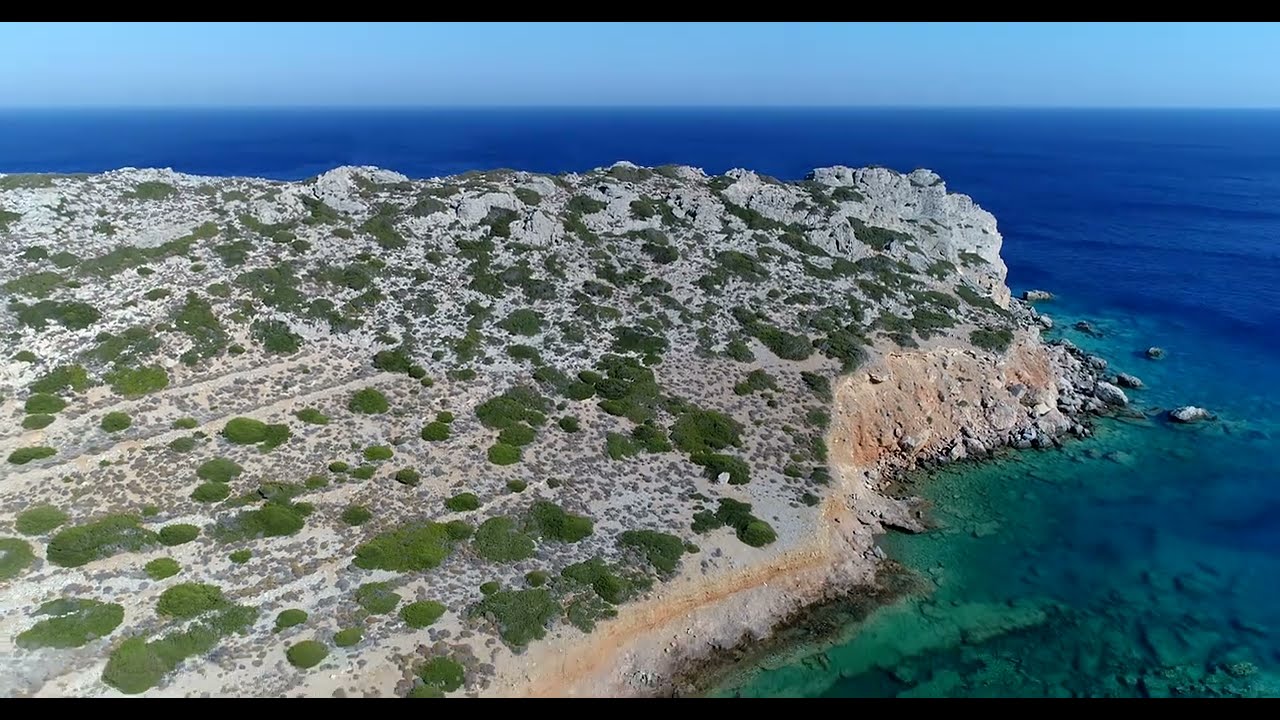The image showcases a dramatic aerial view of a vast gray landmass that abruptly drops off into a vibrant ocean. The surface of the land appears rough and uneven, peppered with circular patches of moss and bushes, which lend it a speckled look, much of it appearing gray rather than green. The cliff face where the land meets the sea displays a gradient of browns, from light brown to dirt-colored hues, transitioning into an emerald green strip right along the edge. This bright green quickly gives way to astonishingly vivid blue ocean waters, which start as a striking electric blue along the shore and darken as they extend further out. The contrast of colors between the equally vibrant blue sky and the unrealistically blue water suggests possible image editing, emphasizing the unusual and almost too-perfect appearance of the scene. Scattered across the gray rock formations, tan rocks provide subtle color variation, complemented by the presence of numerous trees on top of the rocky area.